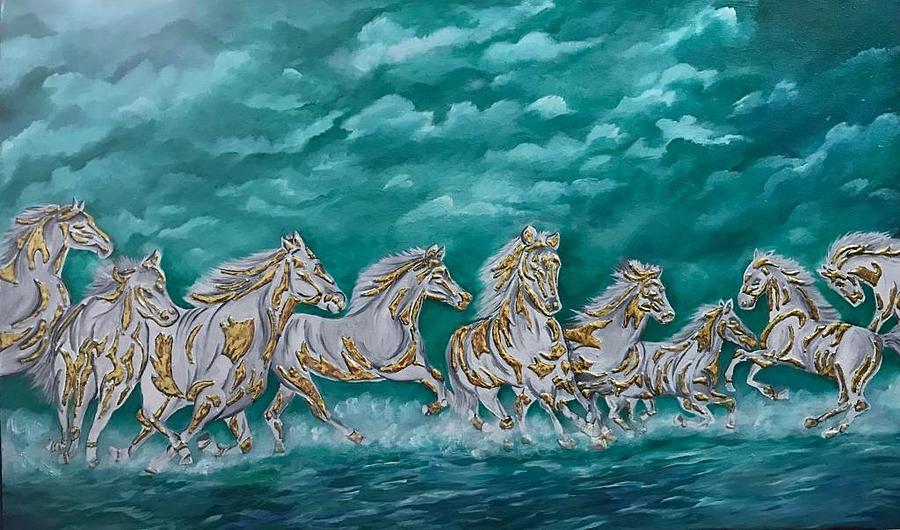The painting depicts a dynamic scene of gray stallions with golden accents galloping across the ocean's surface, amidst a storm. The horses, numbering around nine, are portrayed with a captivating blend of gray, purplish, and whitish hues. Some horses are charging towards the front of the image, while a few appear to be heading in the opposite direction. The setting is enveloped in various shades of blue, from the dark, stormy clouds above to the turbulent ocean below, creating an overall impression of a fierce and tumultuous environment. The sky is filled with blue clouds, ranging from very light to dark hues, especially concentrated in the top left corner. The water beneath the horses is depicted with white-capped shallow waves and splashes, adding to the lively and intense atmosphere of the painting. The composition is long and rectangular, emphasizing the expansive and dramatic nature of the scene.